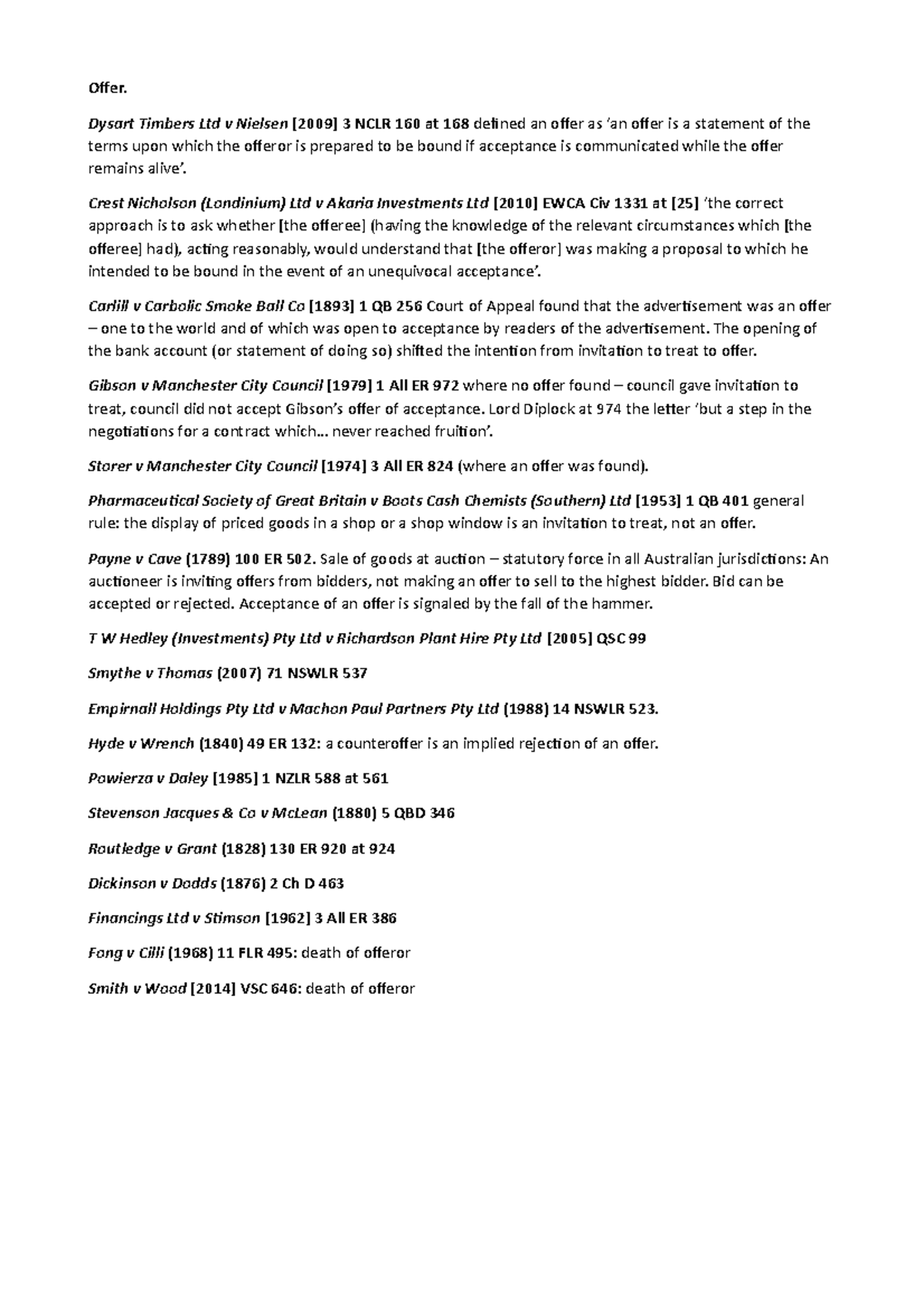### Detailed Caption

Against a stark white background, black text unfolds a series of legal precedents defining the concept of an offer within contract law. The first line reads, "Offer Period," setting the stage for the legal exploration that follows.

The subsequent line references the case "Desert Timbers Limited v. Nelson [2009] 3 NCLRs 160 and 168," where an offer is meticulously defined as "a statement of terms upon which the authority is prepared to be bound if acceptance is communicated while the offer remains alive."

Next, the caption references "Chris Nelson, LTD v. Carrier Investments, LTD [2010]," elucidating the approach to evaluating offers. It states, "the correct approach is to ask whether the offeree, having knowledge of evaluation for exemptions and acting reasonably, would understand that the offeror was making a proposal intending to be bound in the name of unequivocal acceptance."

The historic case "Carlill v. Carbolic Smoke Ball Co. [1893]" is then cited, with the Court of Appeals determining that the company's advertisement was an "offer to the world," open for acceptance through the specified action, thereby shifting the intention from an invitation to treat to a formal offer.

Moving to the case of "Gibson v. Manchester City Council [1979]," the caption quotes that no offer was found because the council merely issued an invitation to treat and did not accept Gibson's offer of acceptance.

In contrast, "Storer v. Manchester City Council [1973]" acknowledges that an offer was indeed found within the circumstances described.

Further, the "Pharmaceutical Society of Great Britain v. Boots Cash Chemists [1953]" case sets forth the general rule that the display of a price list in a shop window constitutes an invitation to treat, rather than an offer.

Finally, "Payne v. Cave [1779]" addresses the sale of goods at an auction. It points out that the auctioneer's call for bids is an invitation for offers from bidders, not an offer to sell to the highest bidder. Acceptance of these offers is signaled by the fall of the hammer, which can accept or reject any bid.

This meticulous detailing of cases provides a thorough insight into the legal interpretations and distinctions surrounding the concept of an offer in contract law.